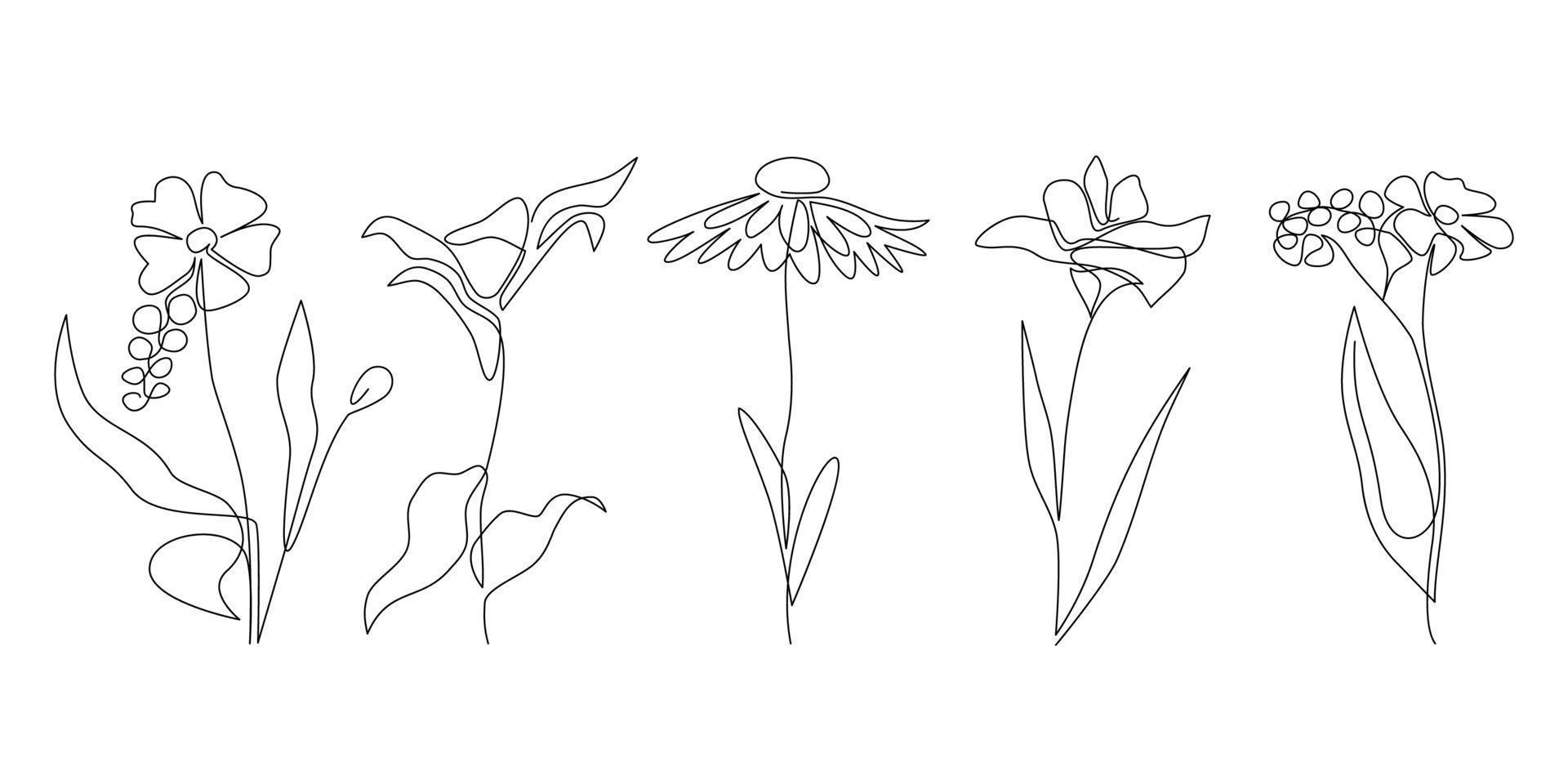This image showcases five black and white line drawings of different types of flowers, arranged in a row from left to right against a white background. Each flower is unique, yet they share a consistent artistic style, with every element—from stems and leaves to petals—crafted from one continuous line of uniform thickness. The flowers are evenly spaced and of similar height, creating a harmonious display. The drawing is both simple and detailed, capturing the distinct characteristics of each flower with minimal strokes, illustrating the beauty of floral diversity with elegant simplicity.